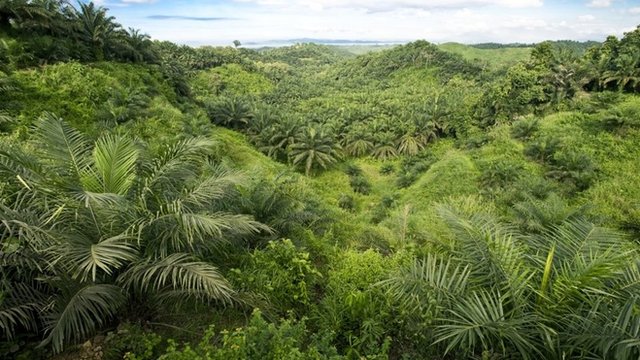An elevated view of a dense tropical rainforest reveals a vibrant, hilly landscape filled with tightly packed treetops in various shades of green. Towering palm trees intermingle with other exotic foliage, creating a lush, uninterrupted canopy. The perspective is from above the treeline, perhaps taken from a mountaintop or a similarly high vantage point. In the far distance, a glimpse of bright blue sky peeks through a scattering of white, puffy clouds, adding a touch of brightness to the verdant scene. The forest stretches out seemingly endlessly, with no signs of roads or buildings, mirroring the untouched beauty of a South African or jungle wilderness. The dense foliage suggests a rich and diverse ecosystem, likely dark and impenetrable at ground level.